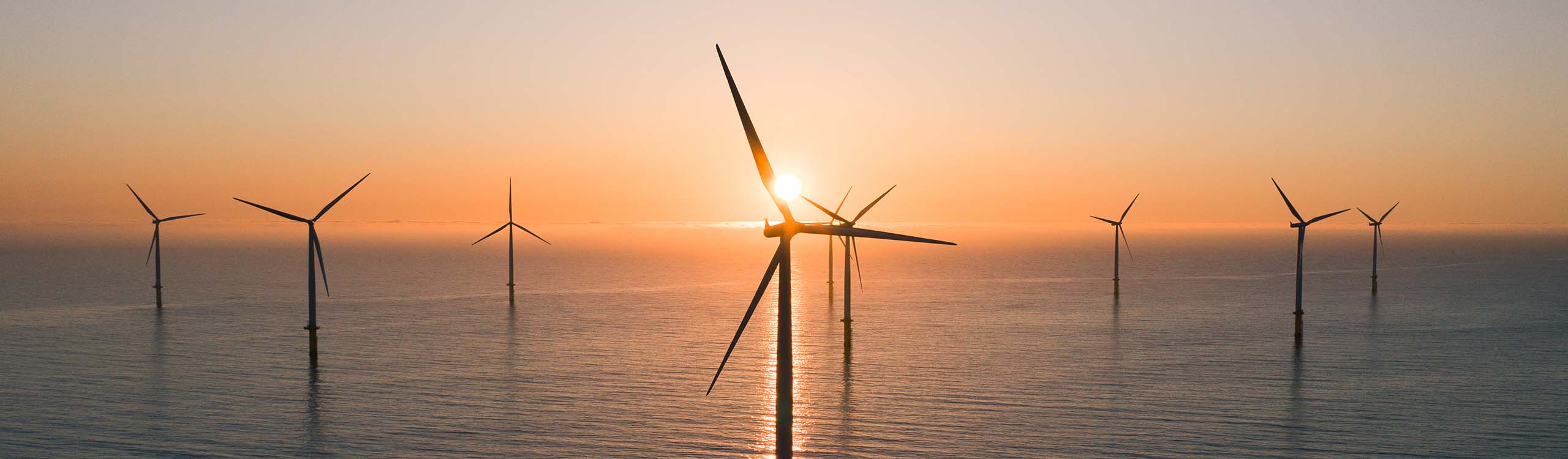In this captivating outdoor photograph, taken either in the early morning or as the sun is setting, the horizon creates a distinct line that beautifully separates the sky and ocean. The vibrant gradient of colors in the sky transitions from a deep blue at the top, through shades of yellow, to a radiant orange near the horizon, emphasizing the sun centered in the image as it sinks towards the water. The calm blue ocean below mirrors the sun's descent, adding a reflective quality to the scene. Scattered across the foreground, six or seven sea-based wind turbines stand tall and still, their three-bladed silhouettes stark against the glowing sky. Three turbines are prominently spaced on either the left or right, with another trio receding into the center, giving a sense of depth. These towering structures emerge straight from the water, their dark forms contrasting sharply with the sunlit backdrop, creating a serene yet striking visual.